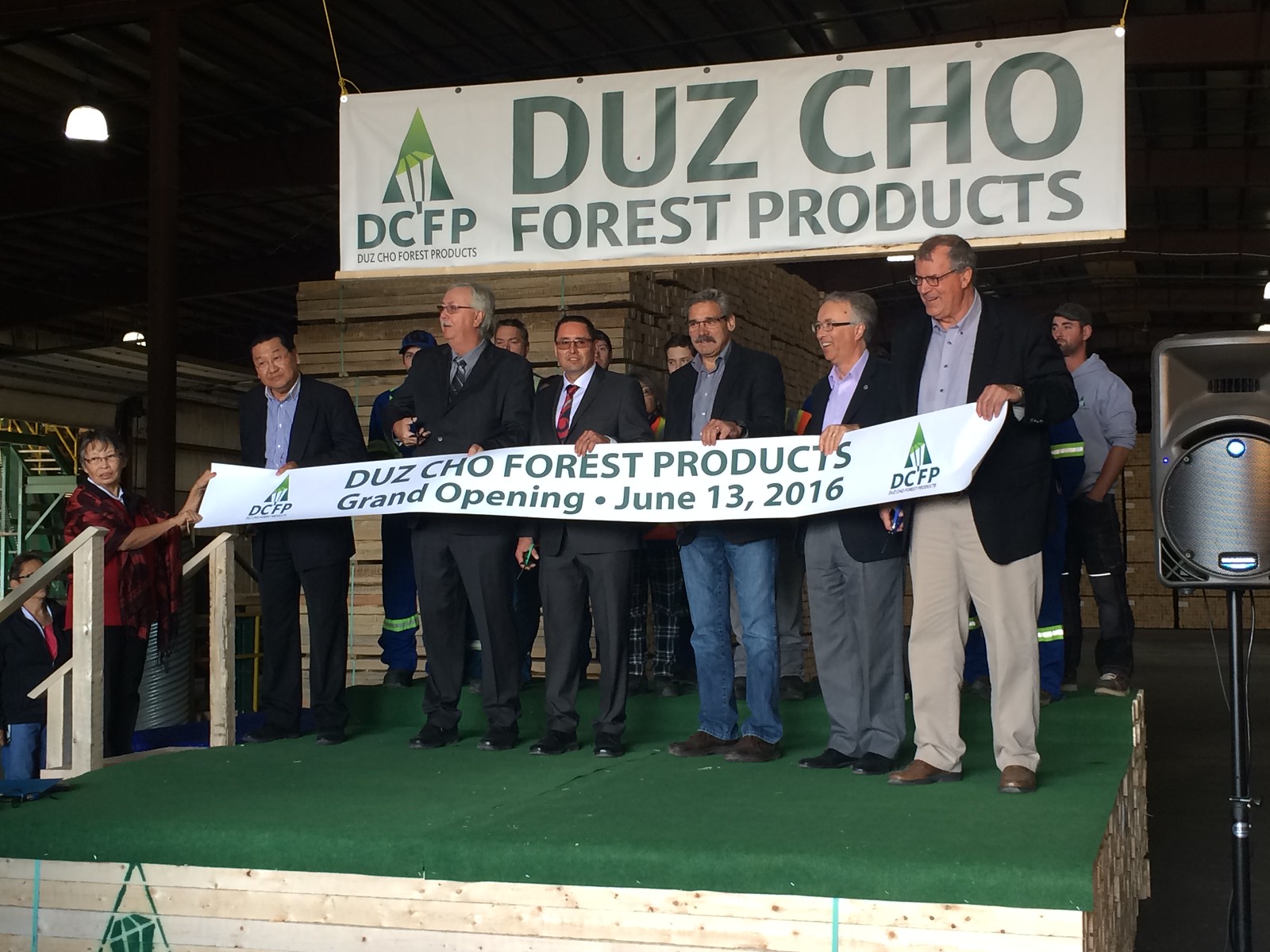The image depicts a grand opening event for Duzcho Forest Products, held on June 13, 2016. Center stage, six men, dressed in a mix of suits, suit coats, and casual attire like jeans and khakis, stand behind a green, wooden platform emblazoned with Duzcho's triangular logo and the initials 'DCFP' in green. These men, appearing to be of diverse racial backgrounds, hold a banner that reads "Grand Opening, June 13th, 2016." To the right, a woman also holds the banner's end. Surrounding the platform are spectators, some visible to the left near the stairs and some in the background. The scene is dimly lit, possibly illuminated by a lamp on the side. The atmosphere suggests an outdoor setting with the green stage symbolizing grass.